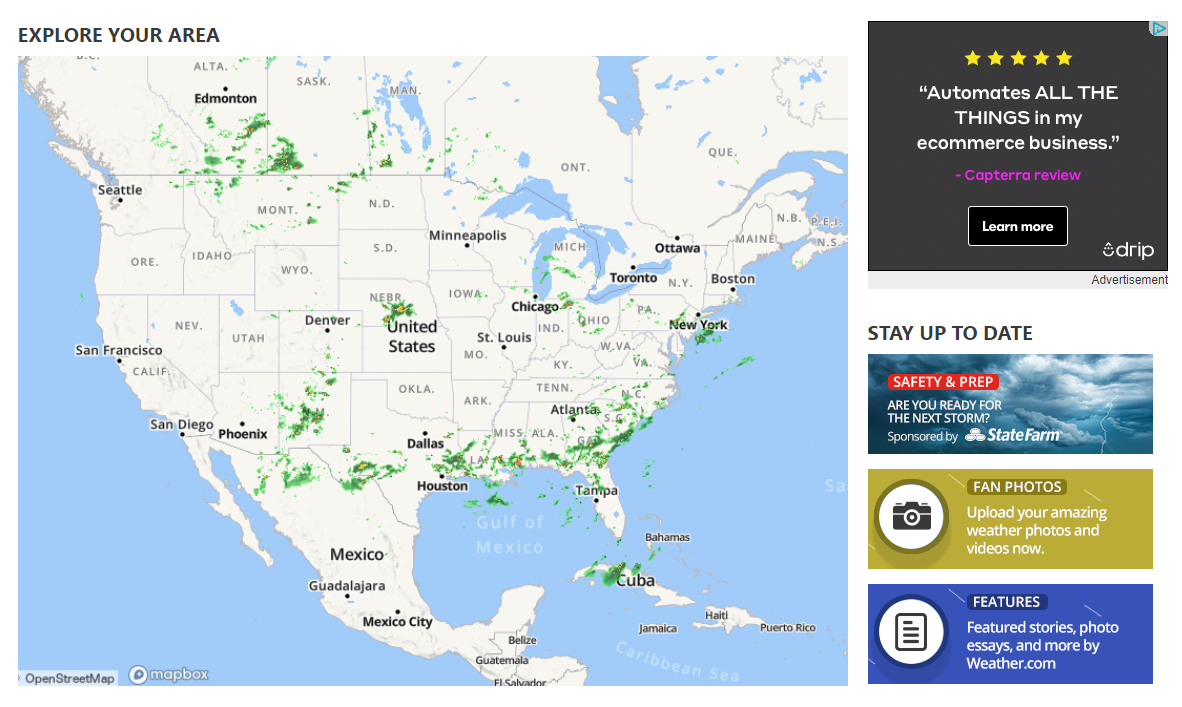This image resembles a map with “Explore Your Area” prominently displayed at the top. The map itself is depicted in white and outlines a triangular area spanning numerous locations. Starting from the top, it lists Edmonton, with Seattle positioned to the left. Moving downward, it includes San Francisco, San Diego, Phoenix, and extends to various cities in Mexico such as Guadalajara and Mexico City.

Within the United States, the map highlights Houston, Dallas, Denver, Minneapolis, Chicago, and then shifts east to Ottawa, Toronto, Boston, and New York. Further south, it notes Atlanta and Tampa, and even stretches to the Caribbean, naming Cuba and the Bahamas. 

On the sides of the image, blue coloration suggests the presence of oceans framing the map. Additionally, on the right side of the image, there are three distinct squares. The first square appears to contain text about automating various aspects of life, possibly related to an e-commerce business. Below this, another square discusses a captured review, and the third square urges viewers to “Stay Up to Date.”